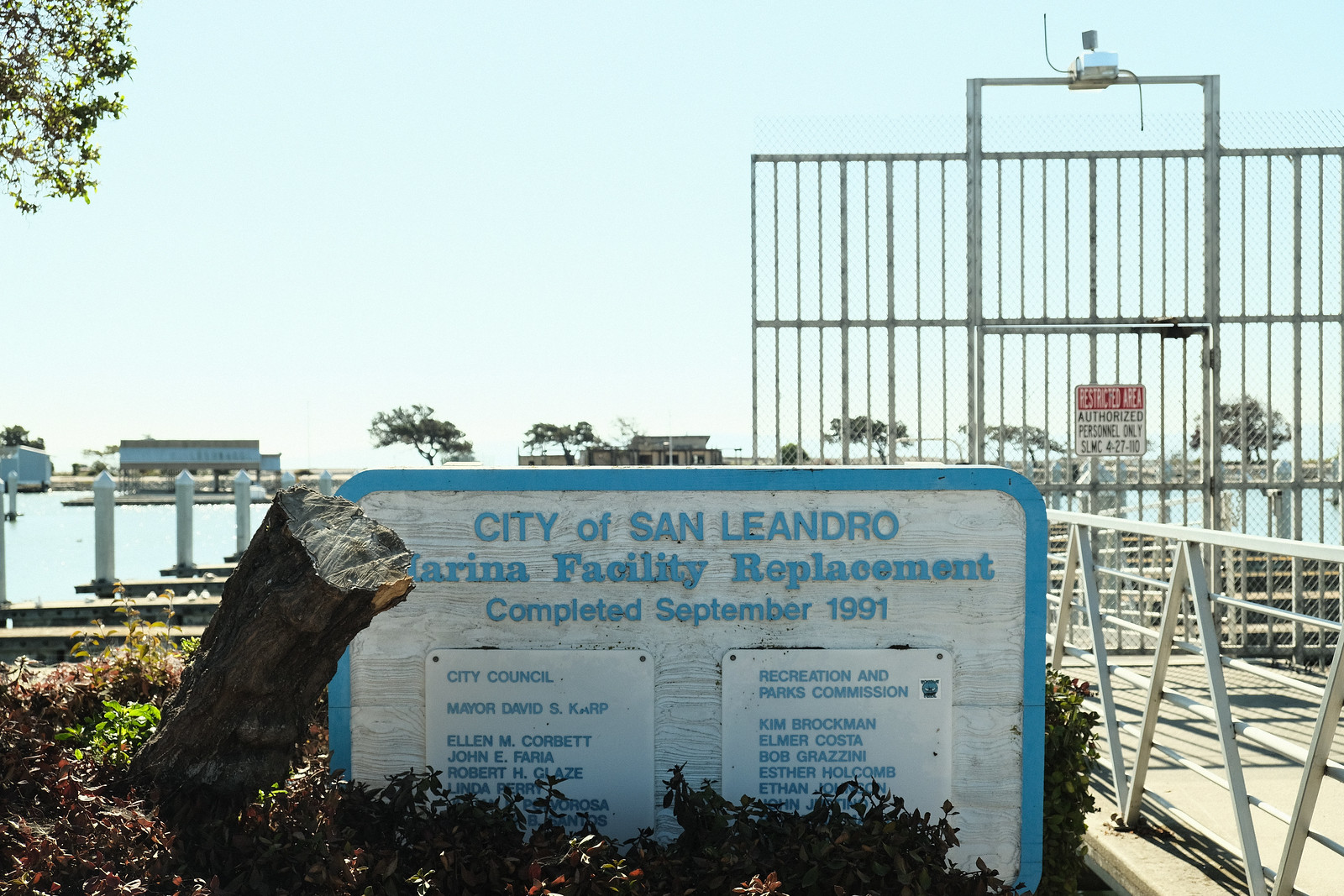This color landscape photograph captures the entrance to the City of San Leandro Marina Facility, framed by a large white sign with a blue border and blue lettering. The sign reads, "City of San Leandro Marina Facility Replacement Completed September 1991," and includes names under "City Council" and "Recreation and Parks Commission." The sign is slightly obscured by bushes and a cut-off tree stump to the left. To the right, there is a tall silver gate with vertical bars and a red sign that states, "Restricted Authorized Personnel Only, SLMC 4-27-10." In the distance, the serene waters of the marina, an iron fence, and a walkway complete the picturesque scene, with buildings and trees visible on the horizon. The aesthetic of the photograph is rooted in representational realism, providing a detailed and accurate portrayal of the marina's entrance.